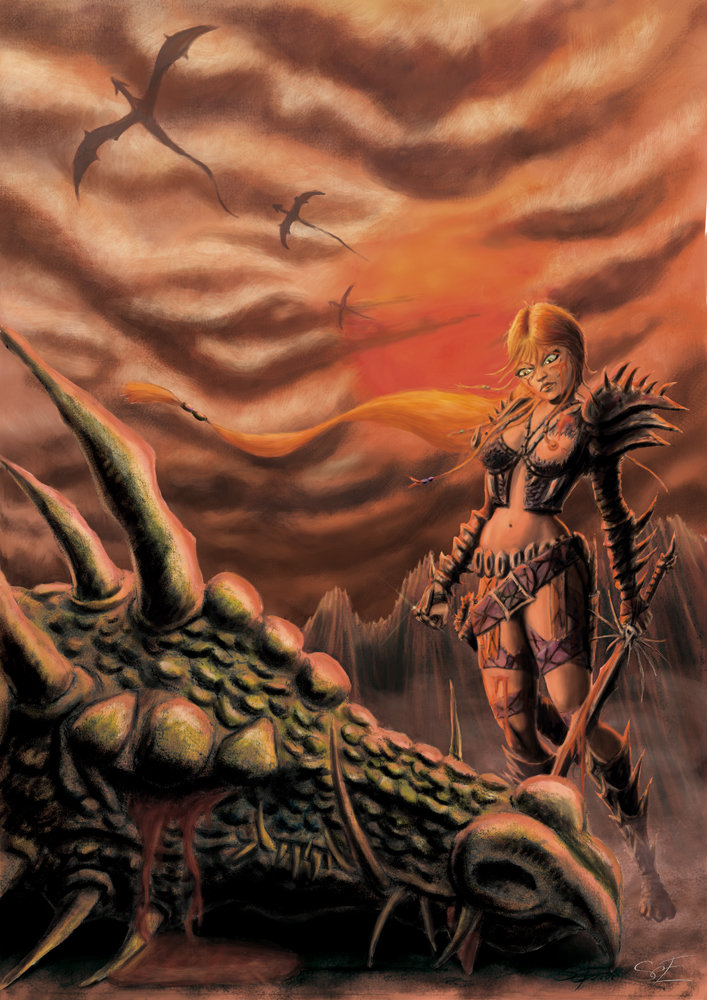This image is a detailed fantasy painting featuring a fierce warrior woman standing over a slain dragon. The warrior, depicted with long auburn hair and wide eyes, wears a revealing metal bikini top adorned with spikes, along with spiked shoulder armor and gauntlets. Her armor is complemented by spiked leather boots. The woman holds an elaborate sword seemingly crafted from dragon scales, with metallic tines near the hilt. Her body bears wounds and scars, including a notable bleeding cut on her cheek, and one breast is exposed from the battle.

The dragon, massive and green, lies with its eyes closed, its head covered in scales, spikes, and horns. Blood streams from its eyes, reinforcing the brutality of the fight. The background is a smoky, murky sky streaked with red hues, filled with silhouettes of flying dragons and rugged mountain spires, evoking a post-apocalyptic, Mad Max-style fantasy world. The warrior’s victorious and solemn stance over the defeated dragon encapsulates the epic nature of the scene.